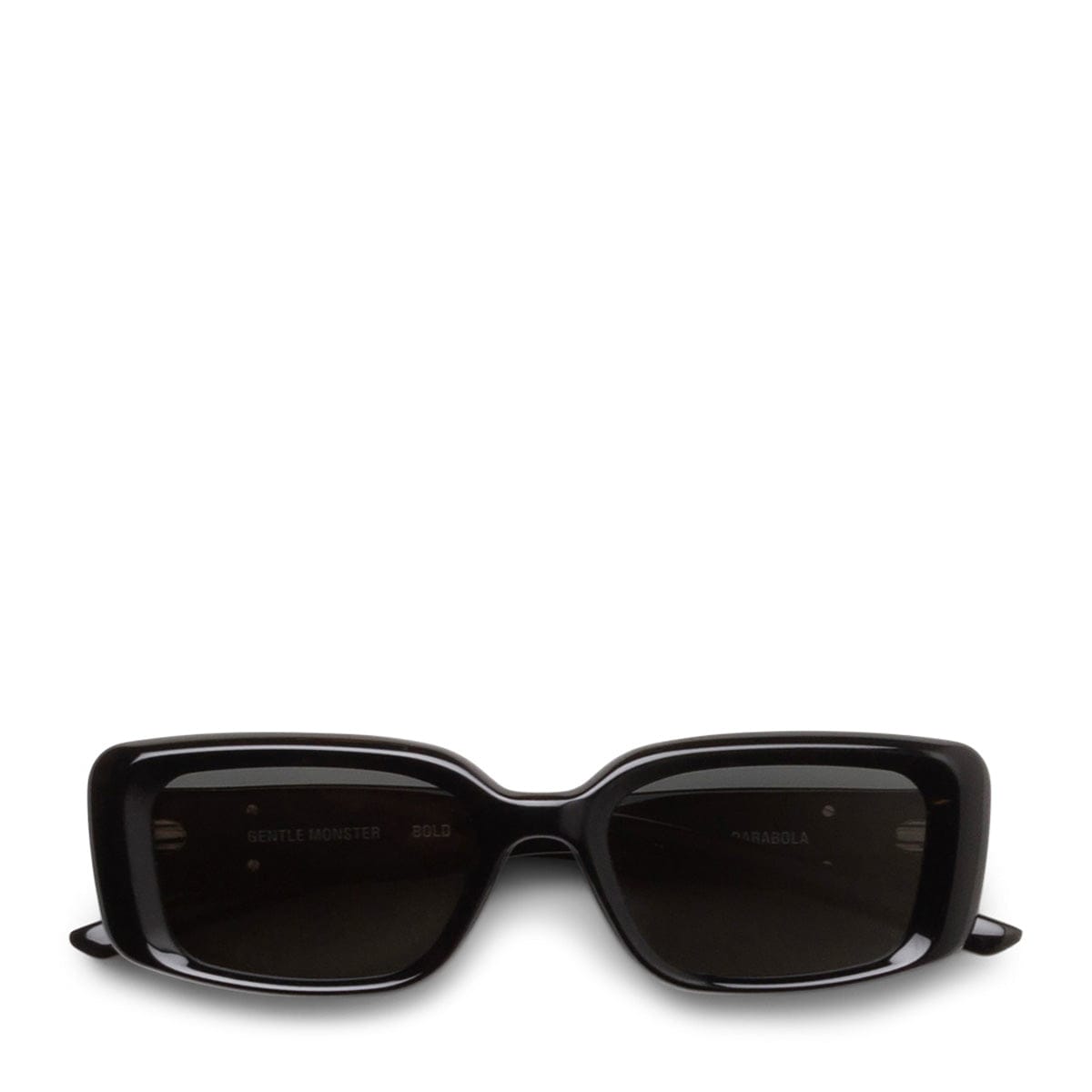The image showcases a pair of black, shiny sunglasses with a simple, sleek design. The frames are predominantly square but with slightly rounded edges, giving them a softer appearance, especially around the nose area where there are no additional nose pieces. The lenses are darkly tinted, yet through their glossy surface, you can perceive the interior. The sunglasses are displayed folded on a white background. Prominent white text is visible on the inside of the ear pieces: "Gentle Monster" boldly appears on the left side, while "Parabola" is inscribed on the right. The frame, which appears to be made of sturdy plastic or fiberglass, is thick and lends a stylish, modern aesthetic to the eyewear.